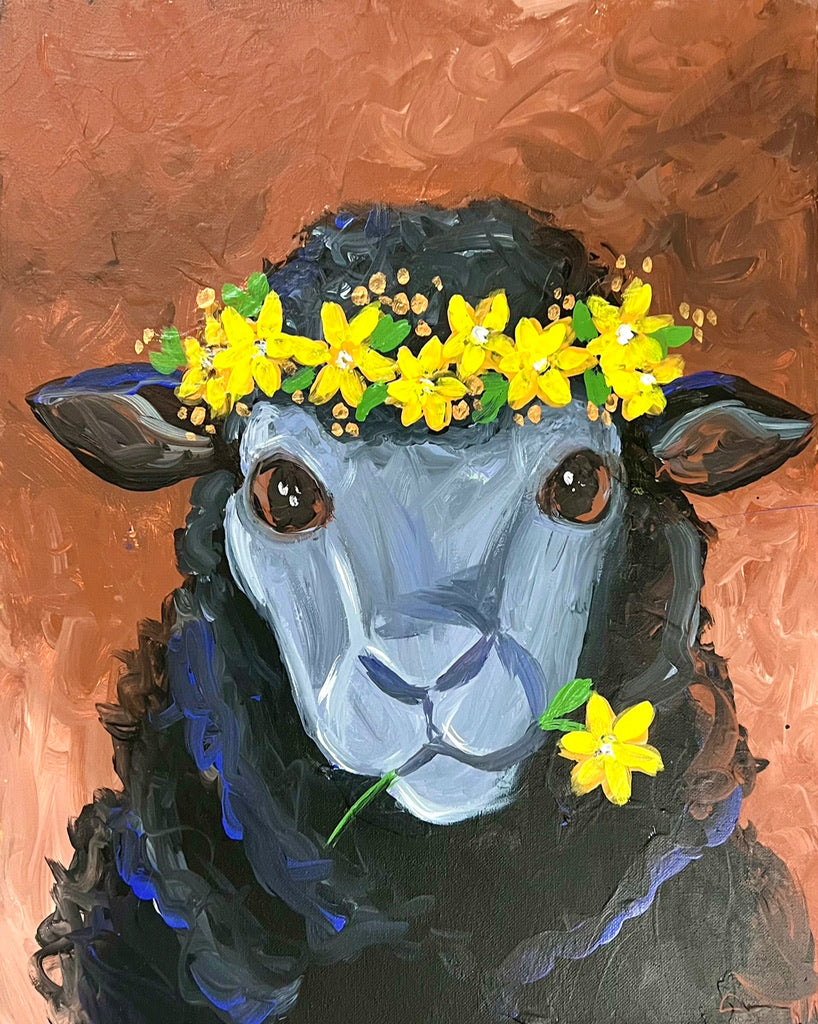This image depicts an oil painting of a black sheep with a close-up perspective, showcasing its serene yet direct gaze. The sheep's face is a light gray, contrasting with its black wool, which is subtly highlighted with blue. It has large brown eyes, with white flecks that simulate light reflections, and black ears slightly tinged with blue, and a mix of gray and brown on the inside. This sheep dons a yellow flower wreath around its head, with each flower detailed with green leaves. In addition, it holds a single yellow flower in its mouth, the stem protruding to one side, and the petals to the other. The background is a rich, dark beige-brown gradient that varies from lighter shades at the bottom to darker tones at the top, offering a textured backdrop where the brush strokes are visible, enhancing the depth and realism of the painting. The sheep's expression is calm and neutral, directly engaging the viewer with its head-on position.